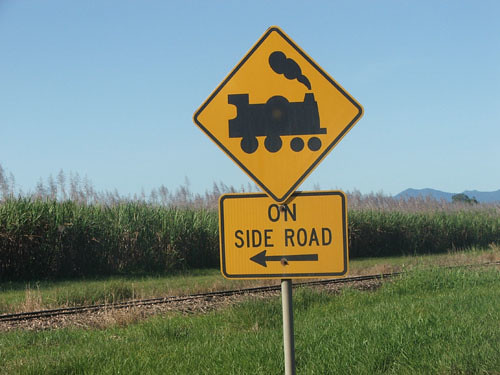In this vibrant country landscape photograph, a prominent yellow diamond-shaped sign with a bold black railroad track symbol alerts travelers to an upcoming crossing. Below it, a rectangular informational sign with a left-pointing arrow provides additional guidance. Framed by lush green grass, the sign punctuates a foreground dotted with wild weeds and the gleaming steel of train tracks that cut horizontally across the scene. Behind the tracks, a vast field of tall corn stretches towards the horizon, swaying gently under the clear blue sky. Anchoring the backdrop, majestic, distant mountains rise against the azure expanse, adding a sense of depth and serenity. The overall color palette vividly blends shades of blue, green, yellow, tan, black, and dark blue, capturing the essence of rural tranquility and rustic charm.